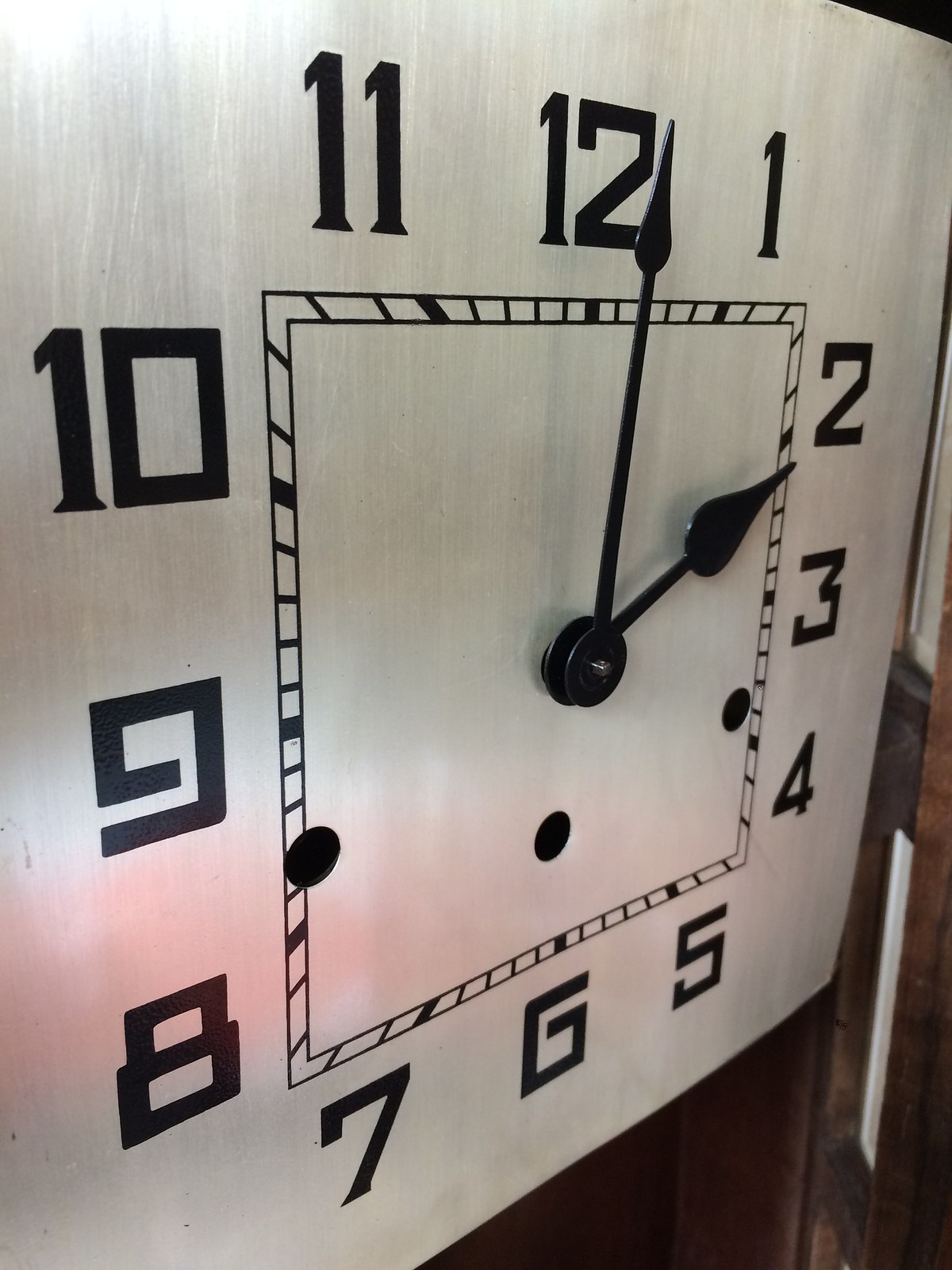A close-up photograph showcases a square clock primarily focused on its face. The clock face is white with subtle, grainy vertical lines that add texture to its surface. Surrounding the face, a hint of the wooden material can be seen at the bottom edge, indicating the clock's mount. The clock numbers, ranging from 1 to 12, are bold and black, prominently displayed along the perimeter. Inside this ring of numbers is a distinctive black, hollow square with four small dash marks positioned between each number. Additionally, dark marks immediately below each number create a visual rhythm. At the bottom of the clock face, three dots are spaced strategically: one centered above the number 6, one near the number 8, and one close to the number 4. The clock hands are positioned to show the time as 2:00, with the longer minute hand pointing directly at the 12 and the shorter hour hand at the 2.